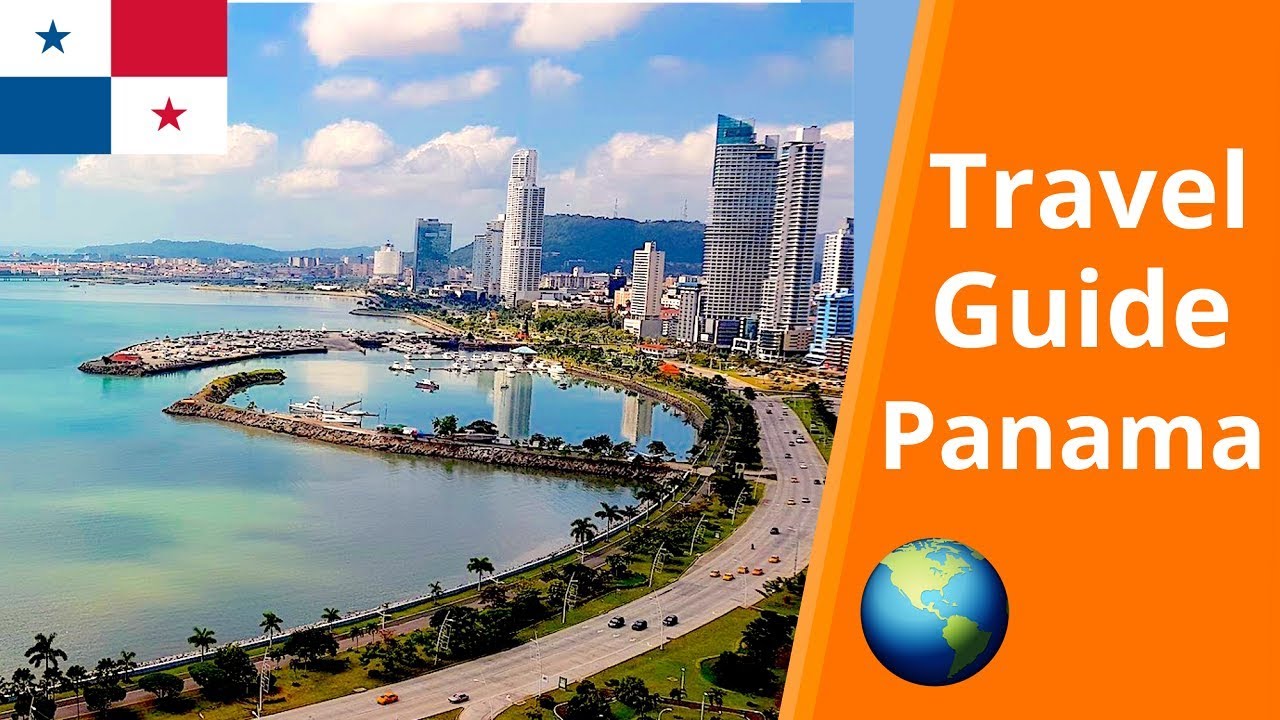In this vibrant image, a striking flag featuring distinct quadrants occupies the upper left corner: a white square adorned with a blue star, a solid red square, a solid blue square, and a solid white square with a red star, respectively. The backdrop is a picturesque panorama showcasing a clear blue sky punctuated with white clouds and an expansive ocean that kisses the shoreline of a bustling metropolis. Towering buildings grace the horizon, juxtaposed against serene mountains, creating a dramatic skyline. The foreground reveals a six-lane highway brimming with traffic, flanked by swaying palm trees. A bridge arches over the roadway while various boats dot the water beneath the azure sky. On the right side of the image, an orange banner reads "Travel Guide Panama" in white text, accompanied by a globe icon. The entirety is bathed in the serene allure of a majestic beachfront, capturing the essence of a scenic and thriving coastal city.